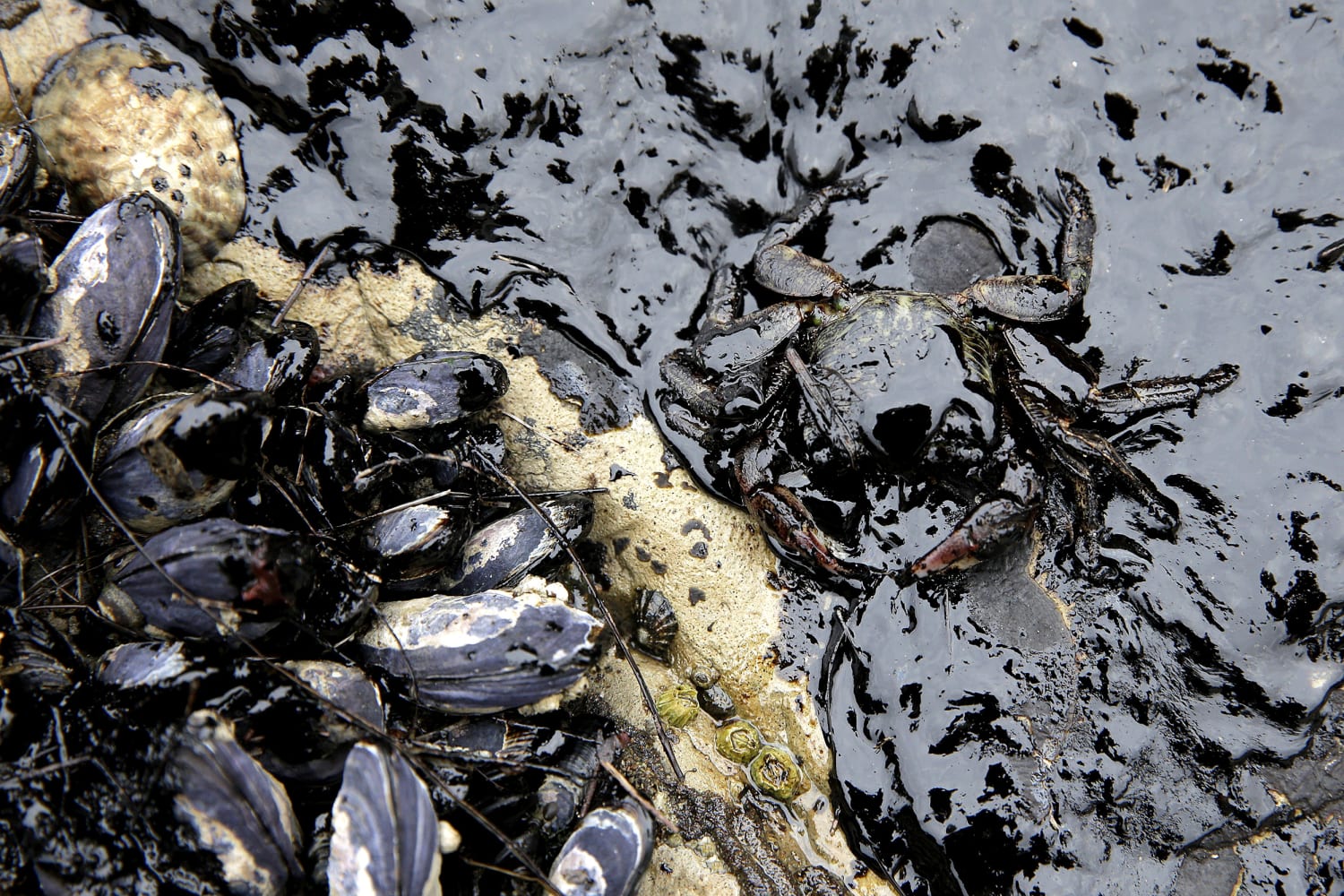This photograph starkly captures the aftermath of an oil spill along a shore. On the left side of the image, a cluster of small, beige clam shells is intertwined with leaves and twigs, stained by patches of black oil. A larger beige shell, partially submerged in the oil, sits atop this heap. A strip of sand separates this amalgamation from the rest of the scene. On the right side, a crab is enmeshed in the thick black sludge, its brownish body with subtle yellow spots and red-tipped claws barely visible through the sludgy coating. The water itself appears sludgy and brown, reflecting a dim shine, engulfing both the crab and the surrounding debris in a grossly viscous trap. The desolate scene portrays the struggle of these small creatures, desperately trying to escape the suffocating slick that envelops everything in its path.